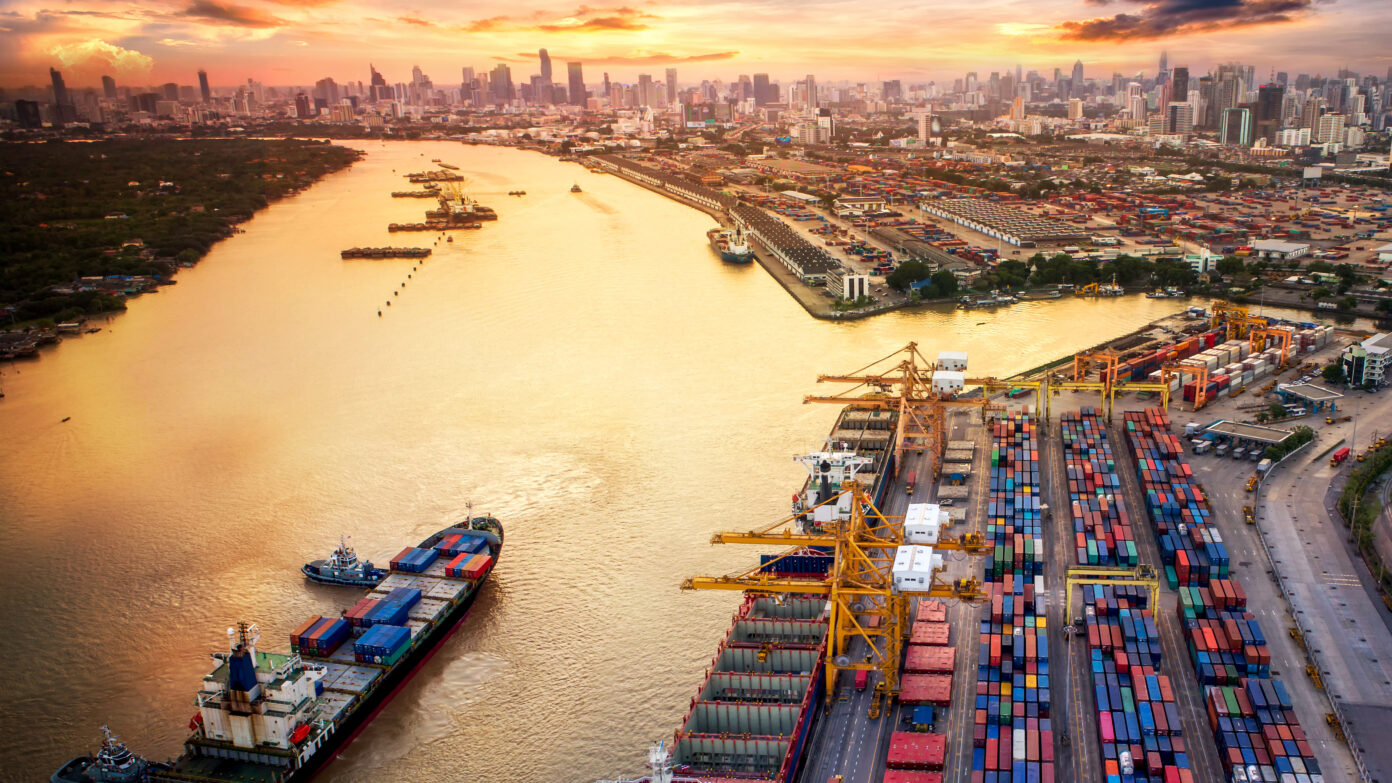This landscape-oriented image, captured from a drone, offers a sweeping aerial view of a bustling seaport assumed to be in New York City. In the foreground on the bottom left, a cargo ship carrying about 12 containers navigates the river, positioned towards the industrial dock area on the bottom right. Here, prominent orange and yellow cranes are actively engaged in unloading the vertically stacked, multicolored containers. 

To the far left of the dock, the river, mirroring the golden hues of the sky, flows alongside low dense vegetation and residential housing. In the background, a vast, distant cityscape with towering gray and purple skyscrapers forms the horizon, setting a stark contrast to the vivid industrial foreground. This intricate scene, captured with photographic realism, is a detailed representation of a dynamic harborfront facility.